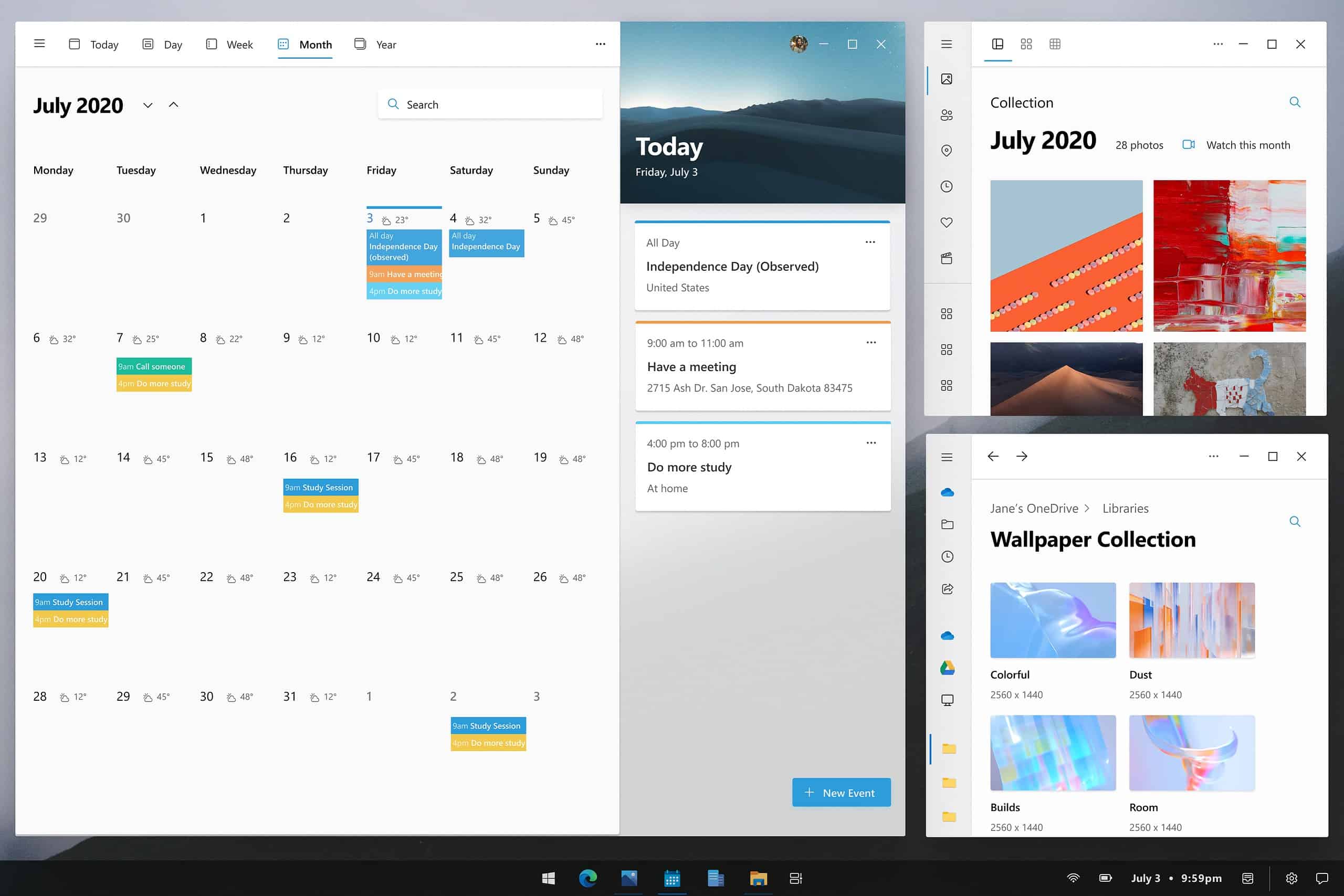Screenshot of a digital calendar interface depicting a detailed schedule for July 2020. This background features a serene image of mountains and a partly cloudy sky. 

Highlighted details include:
- A navigation bar with icons to switch views between day, week, month, and year.
- The current date is displayed as Friday, July 3rd, 2020.
- A search bar with a magnifying glass icon.

Events and information for the selected day (July 3rd):
- An all-day event labeled "Independence Day observed (United States)."
- A scheduled "meeting" from 9 AM to 11 AM.
- Another task listed as "do more study at home" from 4 PM to 8:30 PM.

Monthly view aspects:
- The calendar grid starts with Wednesday as the 1st and ends with Thursday as the 31st.
- Specific dates have colored rectangles indicating events or notes, though some text is indistinguishable.
- July 3rd has notable writing marked within a blue, orange, and light blue rectangle.

Temperature indicators:
- July 3rd: 25 degrees with a sun and cloud icon.
- July 4th: 32 degrees with a sun and cloud icon.
- July 7th: 25 degrees with associated green and yellow rectangle.
- Additional noted rectangles on various dates, including the 16th, with potentially more embedded information.

The interface provides a comprehensive reflection of a daily schedule, temperature forecasts, and key events.